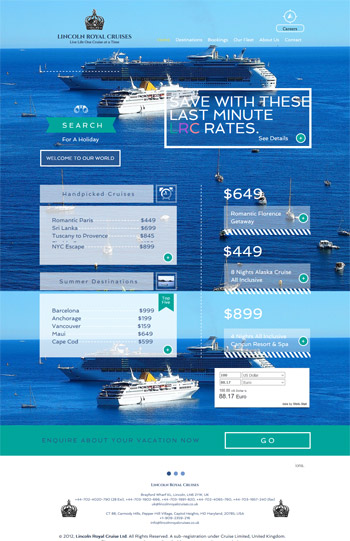**Screenshot Description: Lincoln Royal Cruises Webpage**

The screenshot captures a promotional webpage for Lincoln Royal Cruises. The top of the page prominently features the title "Lincoln Royal Cruises." The background displays a serene ocean scene with two cruise ships: one extremely large ship positioned horizontally and a smaller ship sailing towards it. Scattered across the ocean, several smaller boats add a sense of activity and scale to the scene.

Below the top banner is the main content area featuring various enticing deals and offers. A welcoming message reads, "Search for a holiday. Welcome to our world. Save with the last-minute LRC rate." Emphasizing the availability of exclusive deals, the section lists various handpicked cruise packages with destinations and prices:

- Romantic Paris: $449
- Sri Lanka: $699
- Tuscany to Provence: $845
- New York Escape: $899

A subsequent section labeled "Summer destinations" showcases more holiday options:

- Barcelona: $999
- Anchorage: $199
- Vancouver: $159
- Maui: $649
- Cape Cod: $599

Additional highlights include a “Romantic Florence Getaway” for $449 and an “Eight Nights Alaska Cruise all-inclusive” for $899, though other deal details are blurred and unreadable.

An interactive feature invites visitors to inquire about their vacation plans, highlighted by a white-outlined rectangle labeled "Go." At the page's bottom, there's text too blurry to decipher properly. However, a clear footer notes, "2012 Lincoln Royal Cruise Limited All rights reserved."

This screenshot encapsulates the allure and diverse offerings of Lincoln Royal Cruises, appealing to various travel enthusiasts and highlighting its exclusive, last-minute rates.